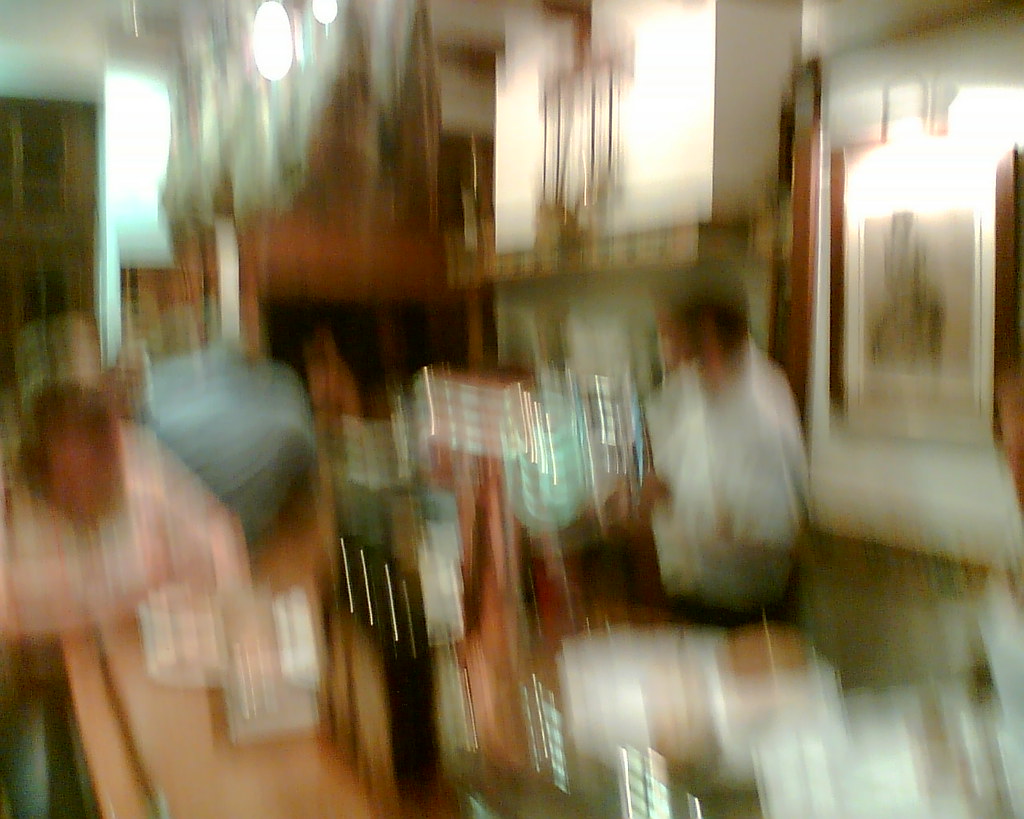This is an extremely blurry photo that likely depicts a bustling bar setting. Dominating the frame is a bar countertop, which appears to be brown, with a mix of clear objects and possibly glasses scattered across it. Behind the bar, there's a person wearing a white shirt and black pants, possibly a bartender, surrounded by various black bottles. The image is imbued with motion blur, suggesting the photographer may have been unsteady, possibly under the influence. In front of the bar, a person in a white long-sleeved shirt seems to be seated. The background features some indistinct wall pictures with light shining on them, adding to the dim bar ambiance. A teal or light blue swirl and a chimney-like structure with a greenish gold ring on the wall, alongside a window in the far corner emitting some light, further contribute to the bar's interior details. Overhead, two light bulbs illuminate the setting, casting a warm glow across this lively yet unfocused scene.